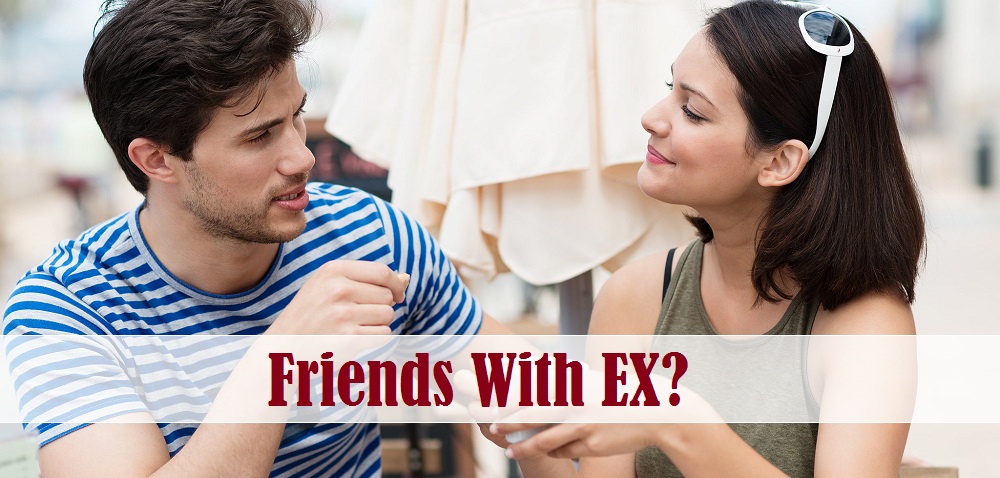The image depicts a scene set at a patio table, featuring a man on the left and a woman on the right, having a conversation. The man, who has black hair and is wearing a blue and white striped shirt, appears to be deep in thought, holding a piece of food in his right hand. The woman, showing keen interest in the conversation, is adorned in white sunglasses with black lenses, a green tank top, and a visible black bra strap over her right shoulder. She has dark hair and pink lips, and she is smiling at the man. They both have white skin. A conspicuous, opaque white rectangle banner stretches across the foreground with the red text "Friends with EX?" prominently displayed, the "EX" capitalized. The background features a white umbrella, lending an impression of a casual, outdoor setting like a beach, poolside, or café. Additional colors in the image include the cream color of the umbrella, which further underscores the relaxed and summery atmosphere.